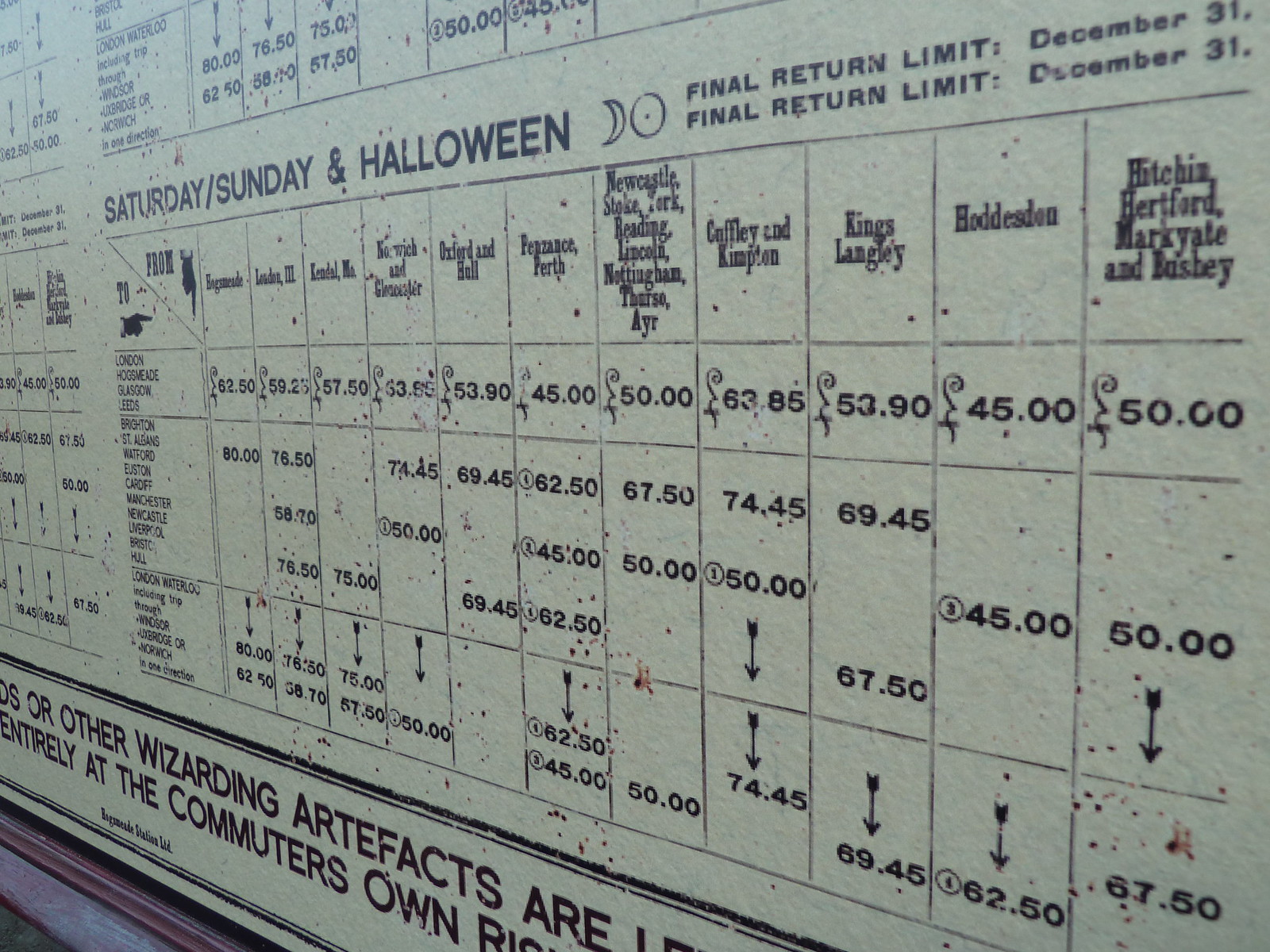The image depicts a large, angled outdoor display or screen listing various types of information, prominently set at about a 30-degree angle clockwise. The top left of the screen features the words "Saturday/Sunday and Halloween" in large black font. Adjacent to this text are images of a crescent moon and a full circle. Directly below this section is the phrase "final return limit December 31st" repeated twice. The board appears to serve a transportation schedule, likely for buses or a similar system, listing names of towns or stops such as Kings Langley, Huddleston, Hitchin, Hertford, Mark, Yate, and Bashie. Under these names, various pricing information is displayed in columns, indicating possible fares for each route. Additional text at the bottom right reads, "or other wizarding artifacts" and "entirely at the commuter's own risk," suggesting a whimsical theme possibly related to a special event or promotion.